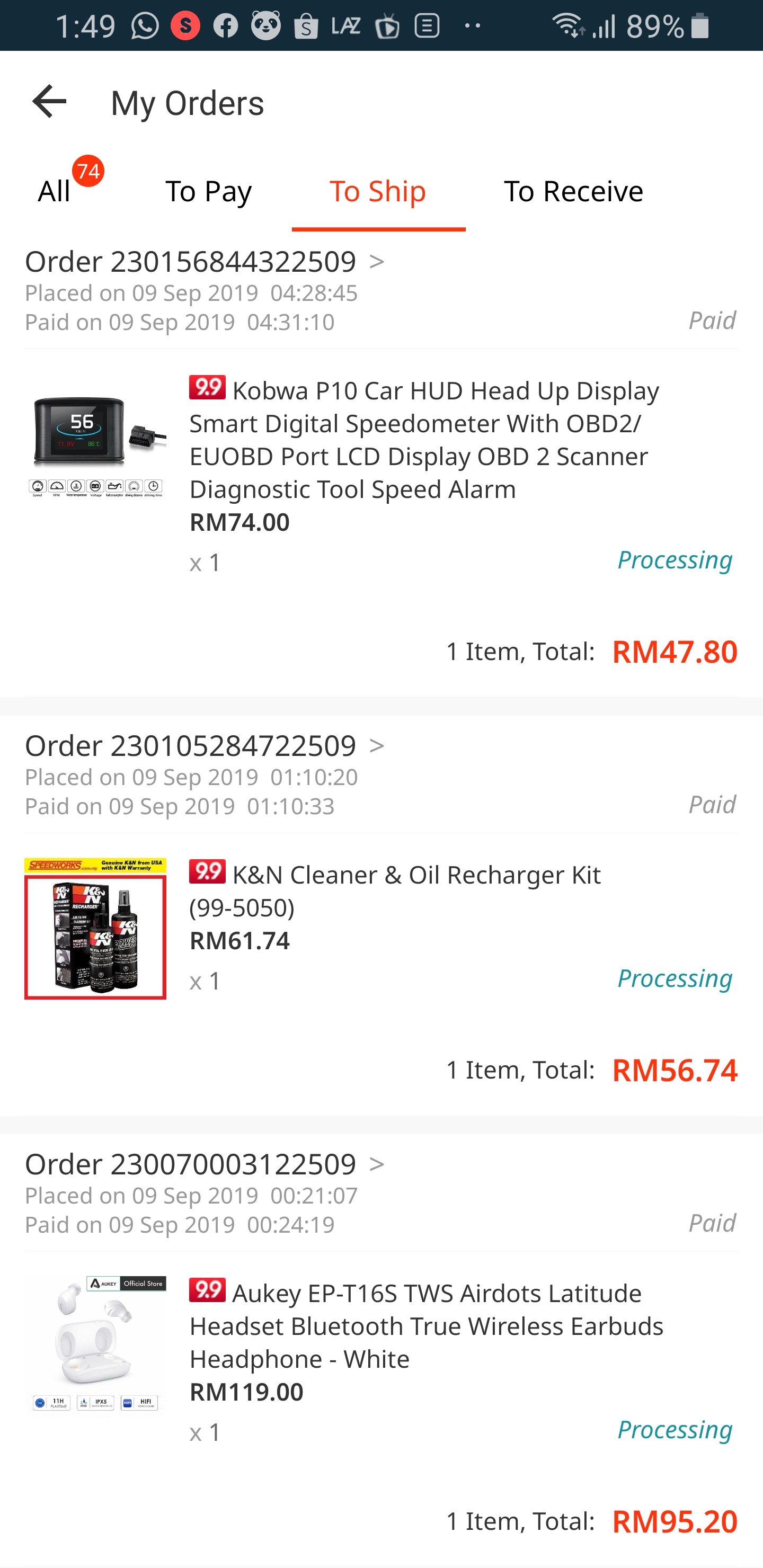The image displays a blurred printout of an order requisition form. At the very top, a black bar showcases the time, "1:49", along with several icons aligned to the right, culminating in an 89% battery indicator.

On the next line from left to right, there is an indicator showing 74 messages. The statuses "To Pay," "To Ship," and "To Receive" are listed, with "To Ship" highlighted in orange, indicating it has been selected.

The following line provides the order number: "230156844322509". The next line specifies the order details: it was placed on "09-09-2019" at "4:28:45" and paid on the same day at "4:31:10".

The order contains three items, though some details are not fully legible. The visible items include:

1. **Kabwa P10 Car HUD Head-Up Display Smart Digital Speedometer with OBD-II**: An image of this item is visible.
2. **KN Cleaner and Oil Recharger Kit**: This item is listed but is not accompanied by an image in the visible portion of the document.
3. **Aukey EP-T16S TWS AirDots Latitude Headset Bluetooth True Wireless Earbuds**: These headphones are white, and there is a faint picture of them to the left of the text description.

Overall, the document outlines the details of an order placed and paid for on the same day, highlighting one of the items being prepared for shipment.